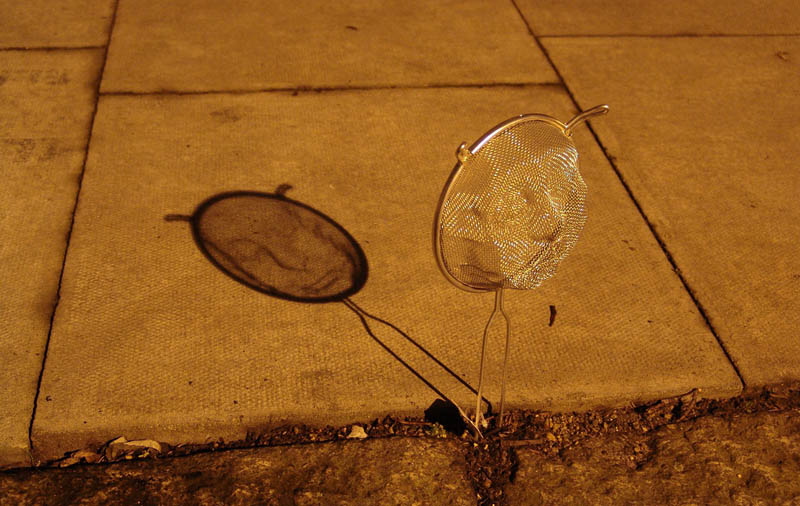In this intriguing nighttime photograph, a small surfboard is captured standing upright on the side of a dimly lit road. The board, bathed in the soft glow of moonlight, casts a peculiar shadow. Interestingly, two prong-like projections extend from the top of the surfboard, resembling bunny ears. Adding to the oddity, the surfboard itself appears to have the outline of a human figure carved into its surface. This detail is mirrored in its shadow, which also curiously forms a human-like face. The surfboard seems to be mounted on a base that vaguely resembles a wheel, though the specifics are unclear. This enigmatic scene, illuminated solely by the lunar light, presents an uncanny visual, as if the surfing figure and its shadow are playfully interacting with the observer’s imagination.